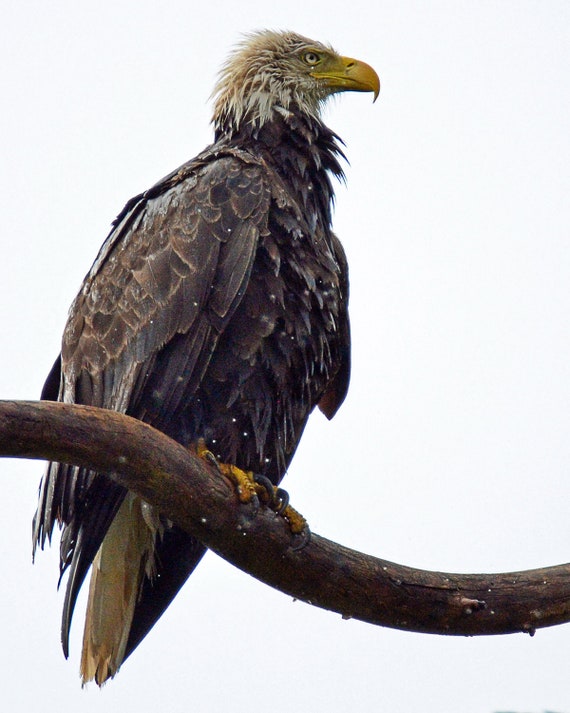In this hyper-realistic drawing, a majestic bald eagle is depicted standing on a branch, set against an all-white background. The eagle's sharp, yellow beak and piercing white eyes with black pupils are striking features. The eagle's head is white but appears weathered and slightly dirty, likely from enduring harsh weather conditions. Its plumage is predominantly dark brown, with some lighter shades of tan, especially noticeable in its wings and chest, which is slightly puffed up. The powerful yellow feet with black talons grip a brown branch that curves down and to the right. Small details, like the white feathers under the back wings and a hint of white on the tail, add depth to this lifelike portrayal of the bird.